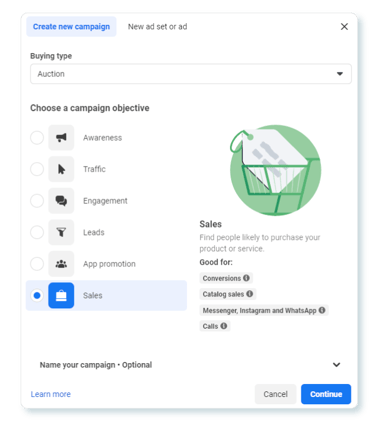The image displays a user interface from a webpage with a clean, white rectangular background. At the top left corner, there is a light blue "Create New Campaign" button with blue text, adjacent to which are the options "New Ad Set or Ad." Toward the right end of this row, a clickable gray "X" allows users to close the rectangle.

Below this header, the section labeled "Buying Type" contains a long, skinny rectangle displaying the word "Auction," with a downward-pointing arrow at the far right for changing the selection.

Further down, a section titled "Choose a Campaign Objective" presents six clickable options. Each option features a gray-bordered white dot, an icon in a square, and corresponding text. The options listed are Awareness, Traffic, Engagement, Leads, App Promotion, and Sales. The "Sales" option is selected, indicated by a blue-dot and blue rectangular highlight. The Sales option also includes a green shopping cart icon with a price tag inside, located off to the right of the word "Sales."